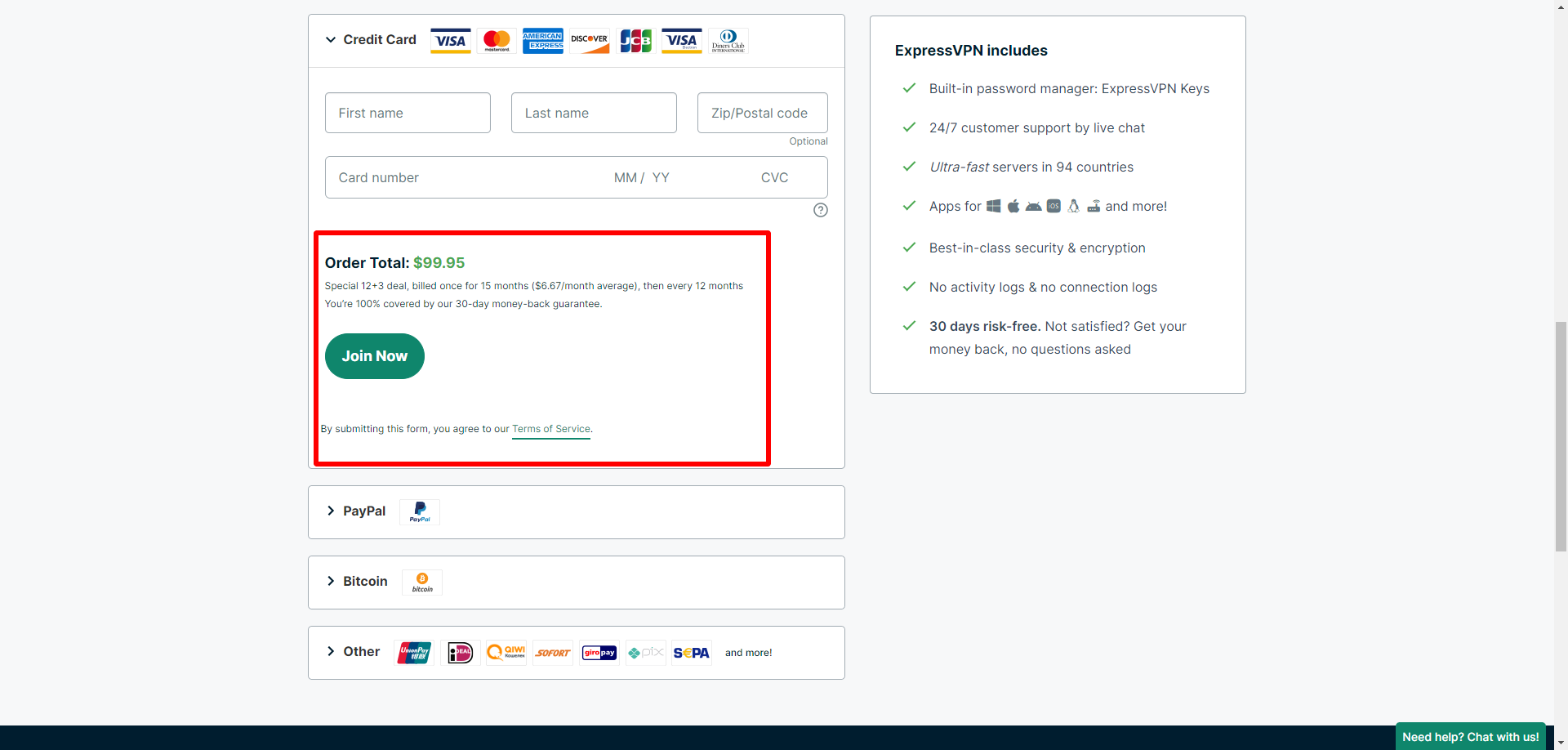This is a highly detailed caption describing the checkout page of a website, presumably for subscribing to ExpressVPN:

---

The checkout page of the website prominently features a dropdown arrow indicating that various credit cards are accepted, including Visa, MasterCard, American Express, Discover, JCB, and Diners Club. A row of three input boxes follows, each containing slightly grayed-out placeholder text for capturing the user's details. The first box is labeled "First Name," the middle box "Last Name," and the right box "Zip/Postal Code (Optional)."

Further down, there is another row for collecting payment information, where users are prompted to enter their "Card Number," the "Expiration Date (MM/YY)," and the "CVC" code.

Below the payment fields, a prominently highlighted red rectangle indicates the order total of $99.95. This section highlights a special 12+3 deal billed once for 15 months, averaging $6.67 per month, with subsequent billing every 12 months. It assures users that they are 100% covered by a 30-day money-back guarantee.

A green highlighted area beneath the order total contains a "Join Now" button in white text. Further down, a row informs users that by submitting the form, they agree to the terms of service, which is underlined in green to indicate a hyperlink.

Near the bottom of the page, icons are displayed for alternative payment methods, including options to "Pay with PayPal," use Bitcoin, and several other unfamiliar cards, each represented by corresponding icons.

On the right-hand side of the page, benefits of subscribing to ExpressVPN are prominently listed, including:
- Built-in password manager, ExpressVPN Keys
- 24/7 customer support via live chat
- Ultra-fast service in 94 countries
- Apps available for Windows, Apple, and more
- Best-in-class security and encryption
- No activity logs or connection logs
- 30-day risk-free trial with a money-back guarantee, no questions asked.